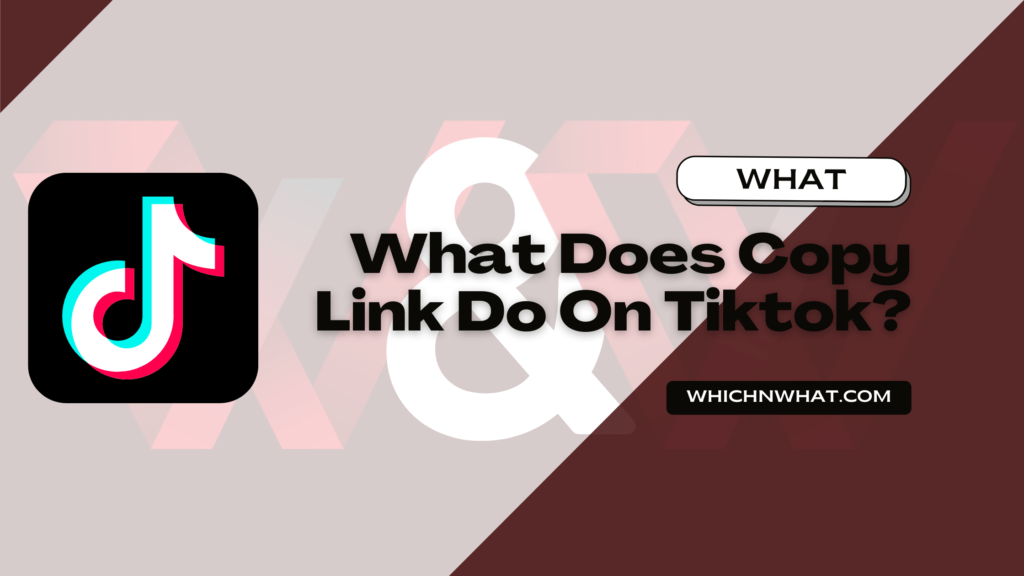This image is a cropped desktop screenshot, showcasing various design elements without revealing the web address, browser, or operating system. In the top left corner, there's a brown triangle, approximately the size of a picture frame, serving as a decorative accent. The bottom right quadrant is dominated by a significantly larger dark brown triangle, occupying roughly a quarter of the image. The background features intricate decorative accents including a gradient 'X,' some ribbons, and an ampersand symbol.

Toward the left side of the image, there's a black square containing a three-dimensional music note outlined in white, bluish-green, and red, identifiable as TikTok's icon. On the right, a white pill-shaped rectangle with an accented shadow beneath, enhancing its three-dimensional appearance, contains the text "what" in black. Below this, another white pill-shaped rectangle displays the text "What does copy link do on TikTok?" 

At the bottom of the image, there is a black rectangle with the words "which and what.com," presumably directing users to a website for further information.